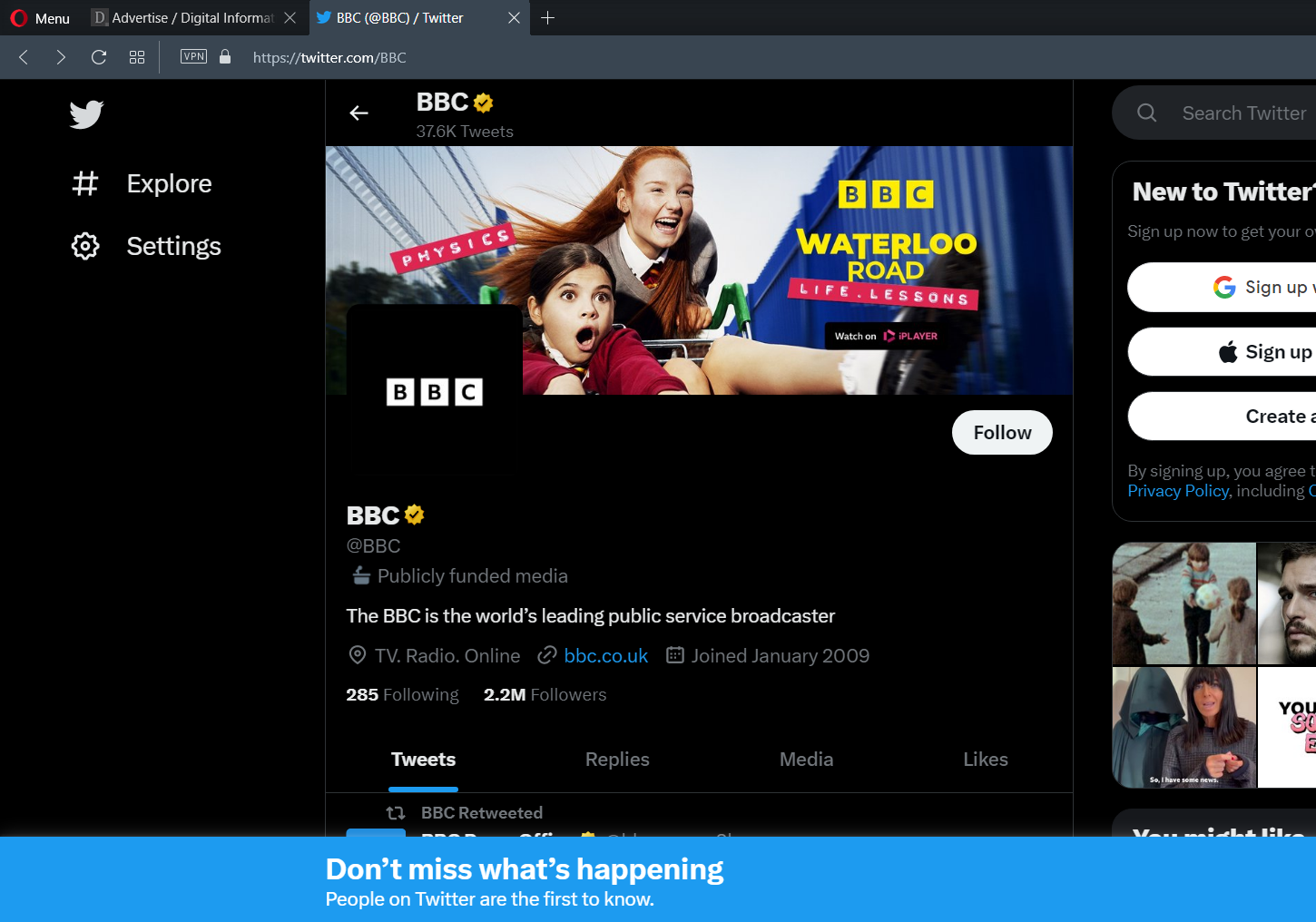The image, a screenshot of a computer screen, features a web browser tab open to a Twitter page, specifically twitter.com/bbc. The Twitter interface is clearly visible with the iconic Twitter bird logo, a hashtag labeled "Explore," and a gear icon representing settings. An arrow pointing to the left indicates navigation, next to which the name "BBC" with a verified checkmark is displayed.

In the main content area, a photo captures two girls running outdoors, with the girl in the front seated in a grocery cart. The girl pushing the cart has auburn hair and a joyful expression, while the girl in the cart has brown hair and appears slightly nervous but is still smiling.

At the bottom of the screen, a promotional banner states, "Don't miss what's happening. People on Twitter are the first to know." Below this, options to "Sign up with Google" or "Sign up with Apple" are presented for new users. Additionally, there is a brief description of the BBC, noting it as "the world's leading public service broadcaster." The entire background of the screenshot is black, providing a stark contrast to the content displayed.